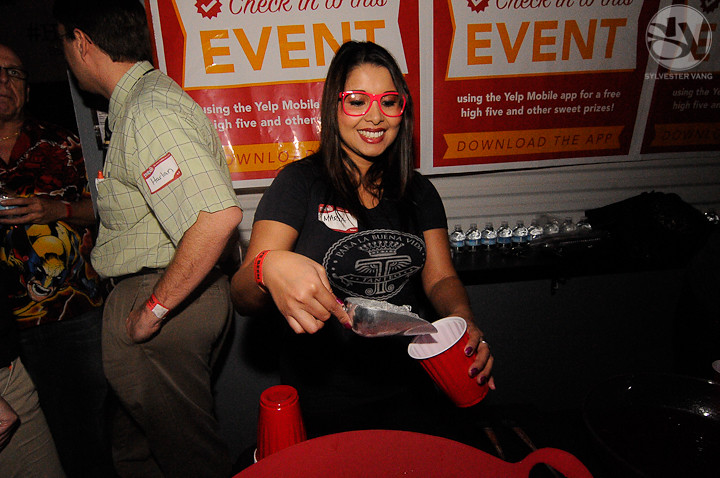Indoors, the photograph captures a bustling event scene centering on two individuals. The woman in the middle, wearing a black graphic short-sleeve t-shirt with a white circular logo and a name tag, is busy pouring ice from a metal scoop into a red and white disposable cup. She sports pink-rimmed glasses, red lipstick, and has brown hair that falls just past her shoulders. In front of her, there’s a large red bowl and more red disposable cups, accompanied by water bottles.

To her left stands a man, identifiable by his tan shirt with a grid of blue vertical and horizontal stripes combined with brown pants. He, too, has a name tag that possibly reads "Harlan." This man is turned away, engaged in conversation with another individual who is only partially visible in the image, identifiable by their intricately patterned shirt. The background features a poster promoting an event, partially readable, stating: "Check in with us event. Using the Yelp mobile app for free high-five and other sweet prizes. Download the app," emphasizing the importance of the app for the event's activities. Despite some of the dimmer lighting, the scene exudes a lively and interactive atmosphere.